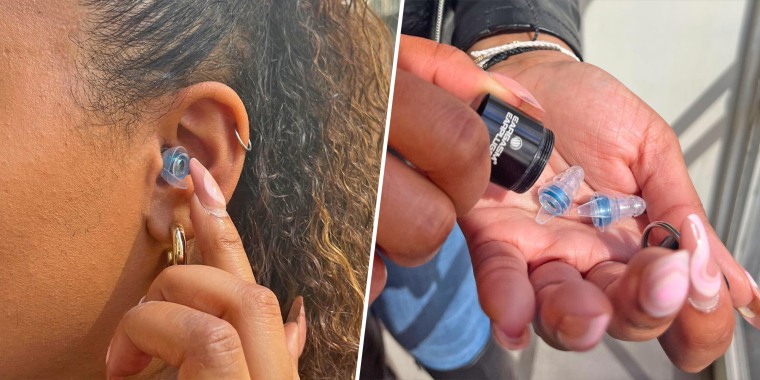This image features a close-up of a brown-skinned woman's ear adorned with two gold earrings and framed by her pulled-back hair. Her manicured nails, painted pink, delicately touch a blue and clear earplug inserted in her ear, suggesting the purpose of sound protection rather than a hearing aid. To the right, the same woman's hands are seen emptying identical earplugs from a black cylindrical container labeled "Eargasm Earplugs" into her palm. The image is captured in a color palette of black, white, gray, brown, clear, blue, and gold. This dual photograph emphasizes both the protective function and design of these earplugs, likely used in noisy environments such as concerts or for sleeping.